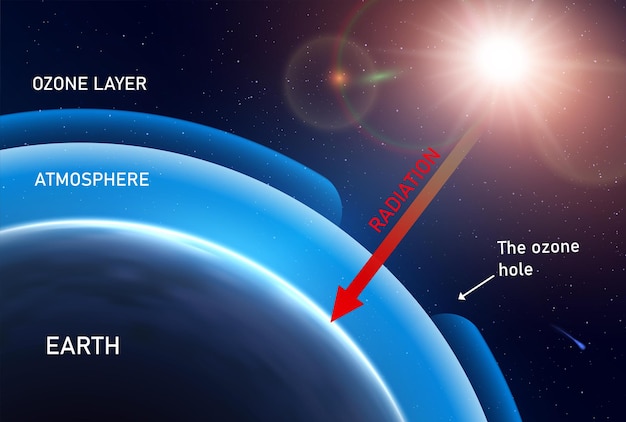This poster is a detailed technical illustration of the Earth and its atmospheric layers, set against a black sky dotted with stars and featuring a streaking meteor in the lower right corner. Positioned in the bottom left corner is a labeled section of the Earth. Surrounding this is a light blue semicircle marked "Atmosphere," which wraps around the Earth. Further out is a dark blue layer labeled "Ozone Layer," with a noticeable gap identified as the "Ozone Hole" in white lettering, accompanied by an arrow pointing to it. In the top right corner, a bright sun shines, casting rays downwards. A prominent red arrow labeled "Radiation" points from the sun toward the Earth, emphasizing the interaction between solar radiation and the planet. The overall composition effectively illustrates the layers of the Earth's atmosphere and the impact of solar radiation, set in the vastness of outer space.